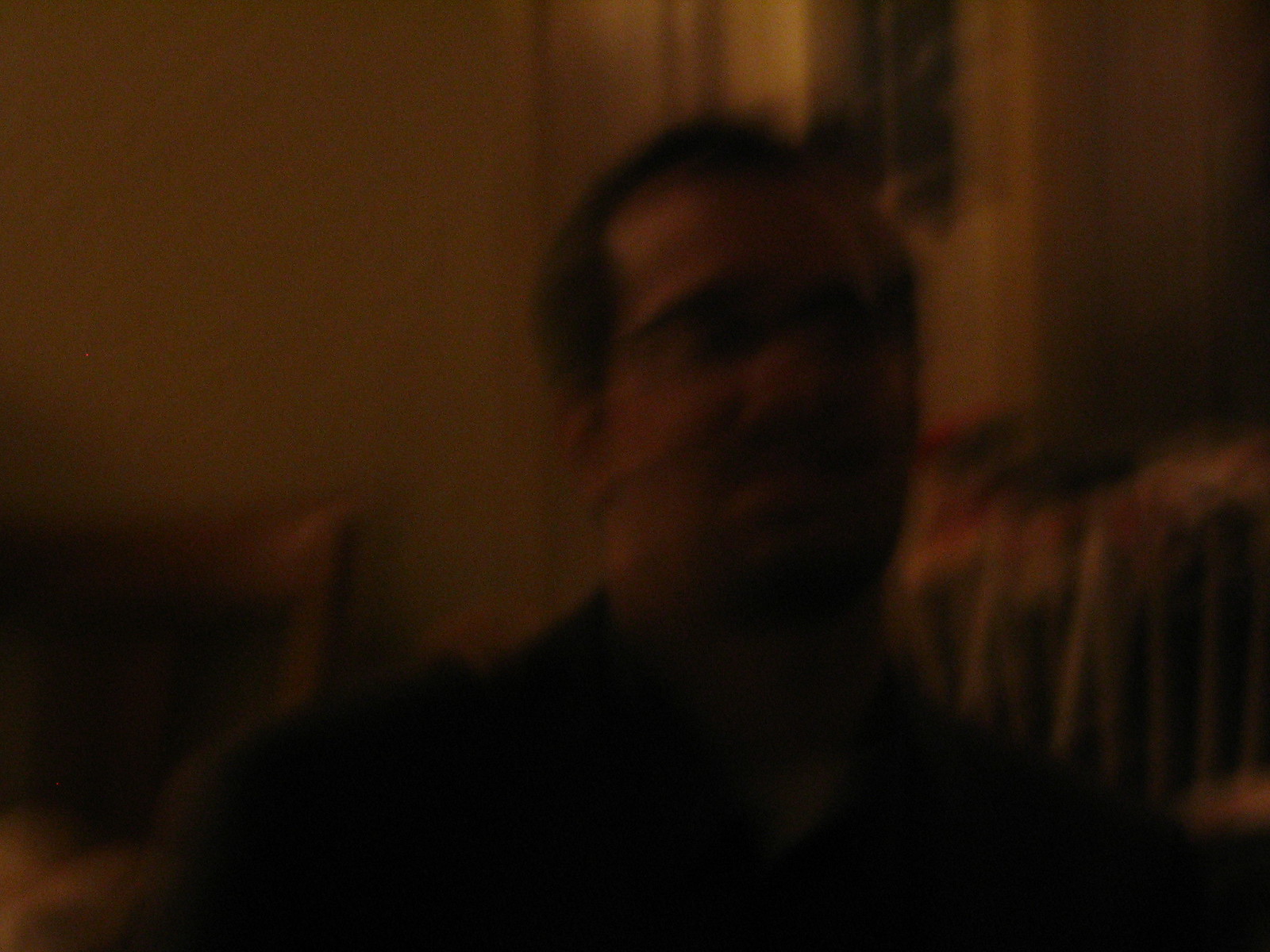The photograph is of very poor quality, making it dark, blurry, and grainy. It appears to capture a man with dark black, fluffy hair and possibly wearing glasses. He seems to be facing the camera, and though the details of his facial features are not clear, he may have a light mustache and goatee. The man seems to be wearing a dark collared shirt, but it’s hard to discern specific details due to the darkness.

The background is indistinct, contributing to the difficulty in identifying specific elements. The wall appears to range from a cream to a light brown or gold tint. There is what seems to be an upright chair visible in the bottom left corner and some sort of wire rack or collection of items that could be sticks or brooms in the bottom right, just above his left shoulder. Above the man's head, there is a white object with black squares that might resemble a window frame at night. Overall, the only discernible details are around his upper body and head, with no clear indications of the environment beyond these fragmented observations.